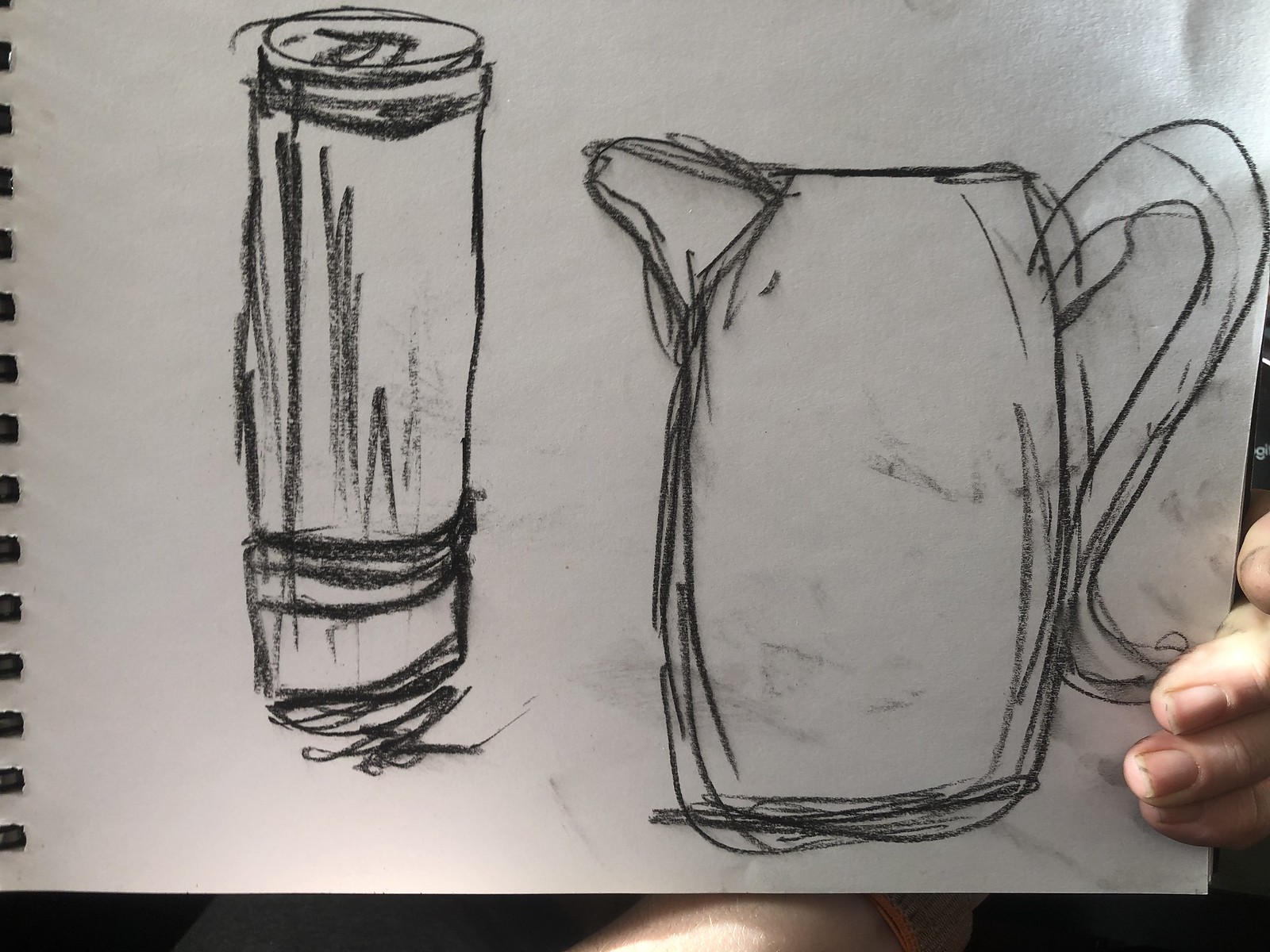A hand-drawn sketch in a black medium, likely chalk or charcoal, is depicted on a white piece of paper held up by a partially visible hand with fair skin and dirty fingernails, suggesting the artist has been working with a black substance. The sketchpad is bound with black rings at the top, with a black backing visible beneath. The main drawing on the right showcases a detailed water pitcher with a pronounced pouring spout and a curved handle. The pitcher has a distinctive cylindrical shape with concave sides, making it wider in the center and narrower at both the base and the top. To the left of the pitcher is a tall, cylindrical object resembling a reusable water bottle. This object features multiple horizontal bands and a scribbled area at the bottom, with additional banding and circular details towards the top, indicating where a screw-on lid and mouthpiece might be.